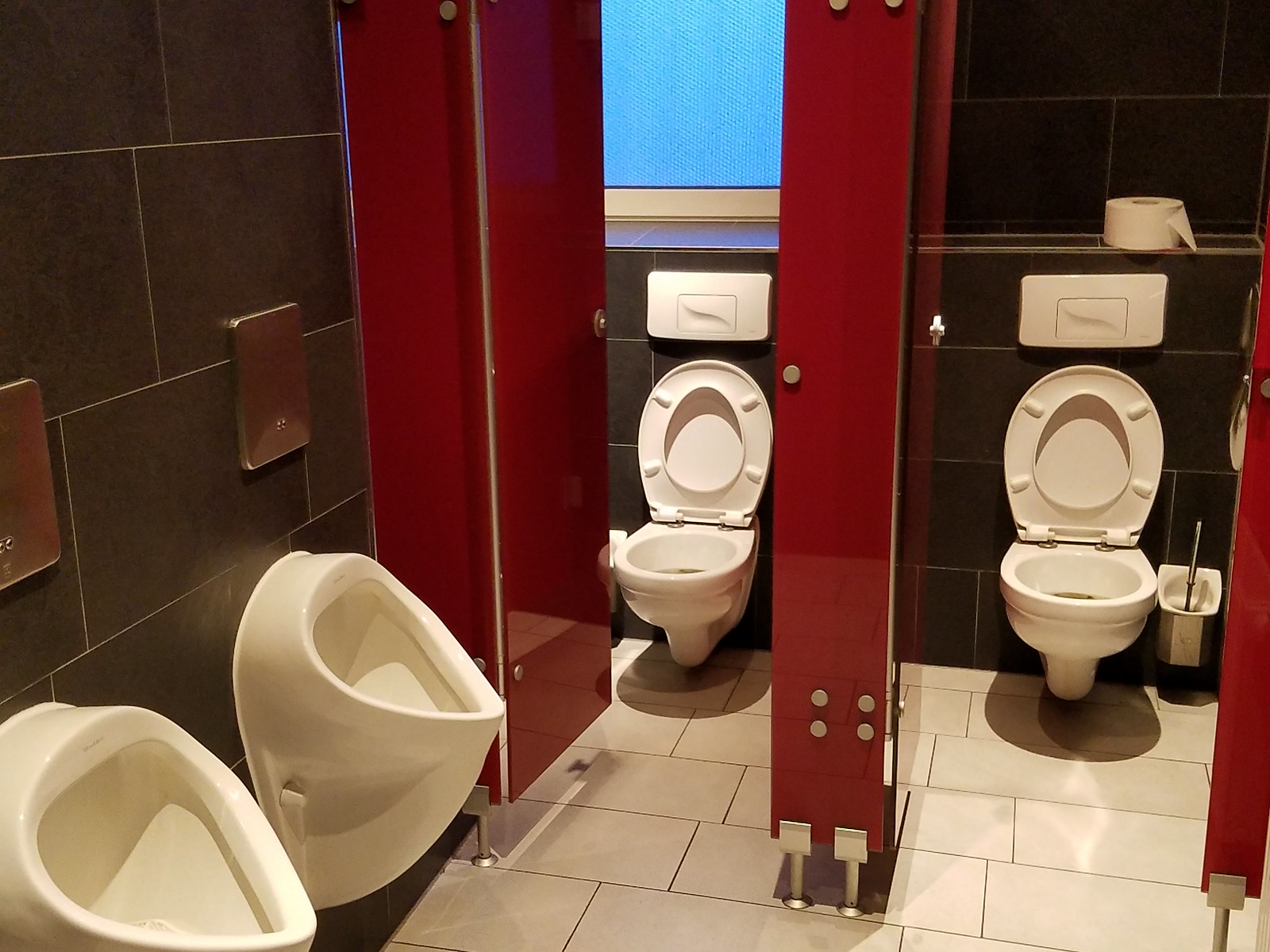This photograph showcases a pristine and potentially luxurious men's restroom, likely situated in a business environment. The restroom features two red stalls, each containing a wall-mounted white toilet with the seat up. Above each toilet, there is a white rectangular box for toilet seat covers. The right-hand stall includes an extra roll of toilet paper positioned on a shelf above the toilet, and both stalls have a cleaning brush conveniently placed beside the toilets. The room’s walls, adorned in dark brown or black tiles, contrast sharply with the sleek, white tile flooring. 

On the left side of the image, two modern-style, white urinals are mounted against the dark tiled wall, each equipped with a gold or silver flush valve directly above them, which likely contain sensors for automatic flushing. These urinals are notably clean and lack handles for manual operation. The restroom also features contemporary nickel-plated hardware on the stalls, enhancing its modern appeal. There’s no divider between the urinals, and the cleanliness of the entire setup suggests a higher-class public restroom. The overall scene is softened by a large blue opaque window above the central area, which casts a subtle blue light, adding to the aesthetic without compromising functionality.